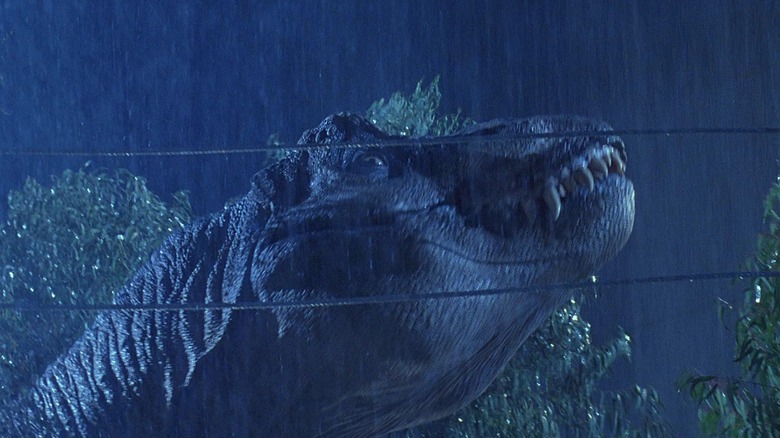This image is a striking screencap from the iconic scene in the original 1993 film *Jurassic Park*, directed by Steven Spielberg. It captures a dark, tense moment as the Tyrannosaurus Rex (T-Rex) approaches the metal wires of an electric fence at night. The landscape orientation frames the scene with the shorter sides on the left and right, and it's shrouded in darkness, hinting at the dense atmosphere of the movie's horror elements. The T-Rex is seen in a detailed profile shot, its mouth slightly open to reveal sharp teeth and a piercing eye, emphasizing its menacing presence. Two taut, horizontal wires pass in front of the T-Rex, marking the boundary of the fence, while foliage and trees are subtly visible in the background, particularly in the lower right-hand corner and around the middle left above the T-Rex's head. The overall composition of the image is memorable, evoking the suspense and groundbreaking special effects that made *Jurassic Park* a landmark in cinematic history.